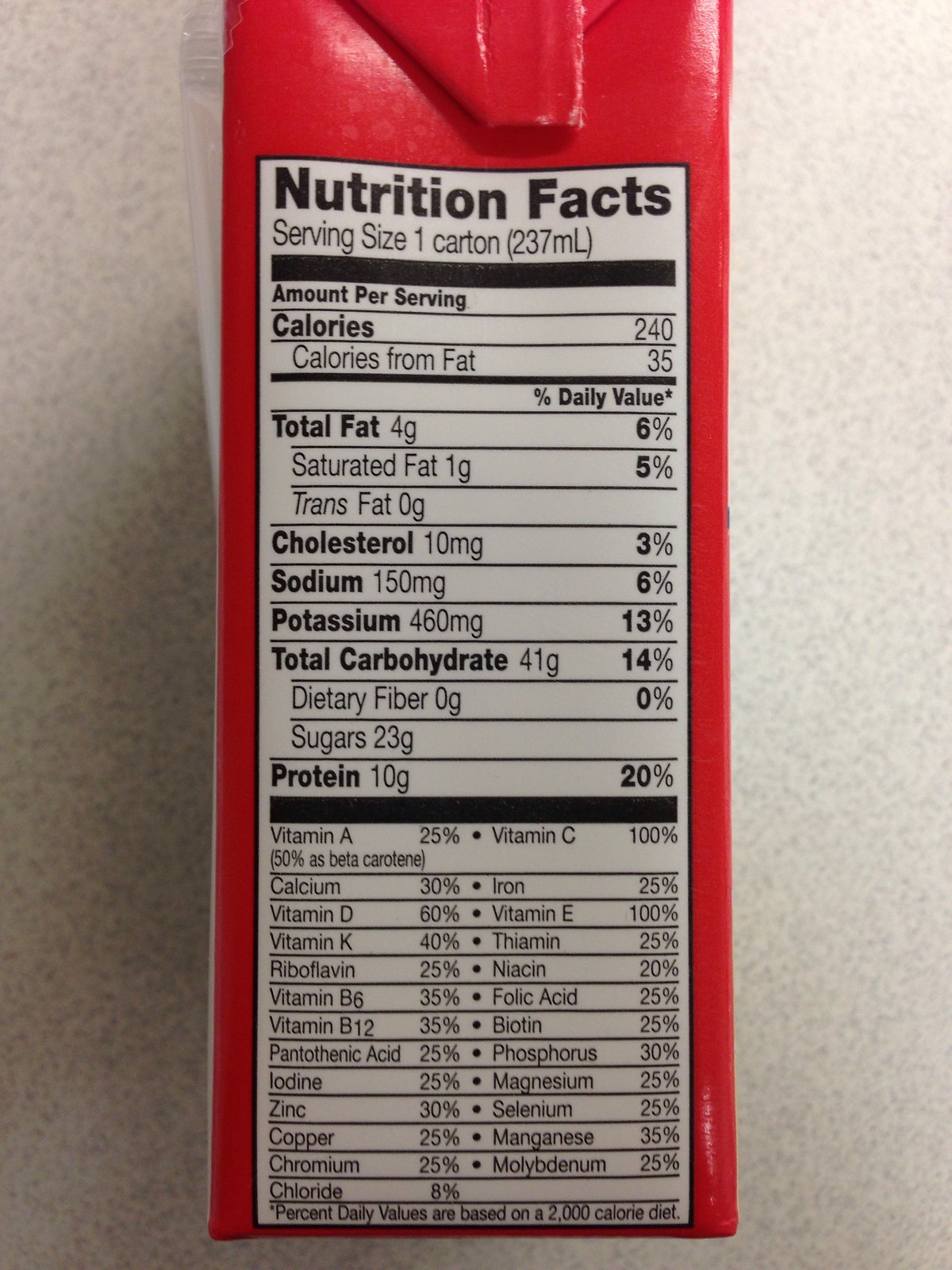On a sleek, white granite table, there's a juice box prominently displayed, with its nutrition label facing the camera. The label details the nutritional content: each 237 ml serving contains 240 calories, including 35 calories from fat. The total fat content is 4 grams (6% of the daily value), with 1 gram of saturated fat (5%) and no trans fat. It also lists 10 mg of cholesterol (3%), 150 mg of sodium (6%), 460 mg of potassium (13%), 41 grams of total carbohydrates (14%), including 0 grams of dietary fiber (0%) and 23 grams of sugars. Additionally, the juice box provides 10 grams of protein, which is 20% of the daily value.